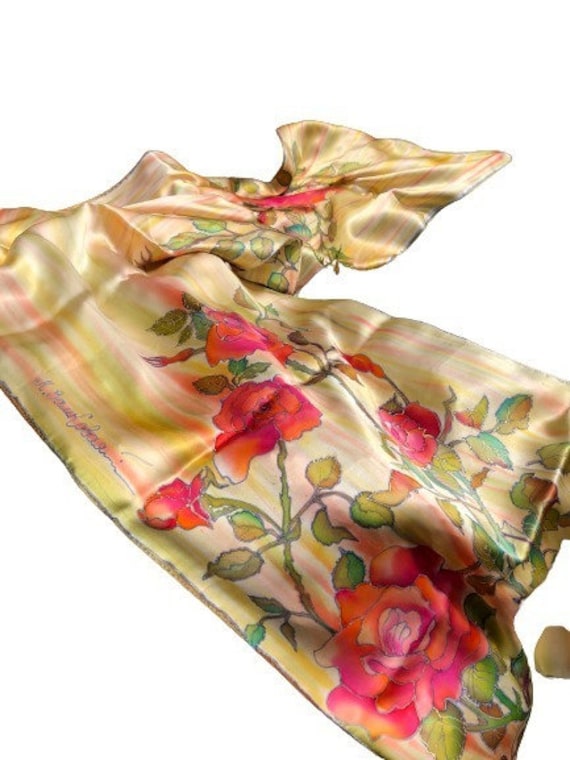The image showcases an elegant, silk scarf adorned with a stunning floral motif, featuring prominently red roses in full bloom, accompanied by lush green leaves. The base of the scarf is a golden hue, accented with streaks of yellow, red, and orange, lending a vibrant watercolor-style aesthetic. The fabric's surface is shiny and delicate, creating a luxurious appearance. The pattern starts larger at the bottom and gracefully snakes upward along the length of the scarf. The scarf itself is slightly wrinkled, adding texture to its presentation. A unique detail is the artist's signature in blue ink along the bottom edge, hinting at its hand-painted, one-of-a-kind nature. The scarf's blend of gold, cream, red, orange, pink, and greens, with touches of blue-green, makes it a beautiful and fashionable accessory.